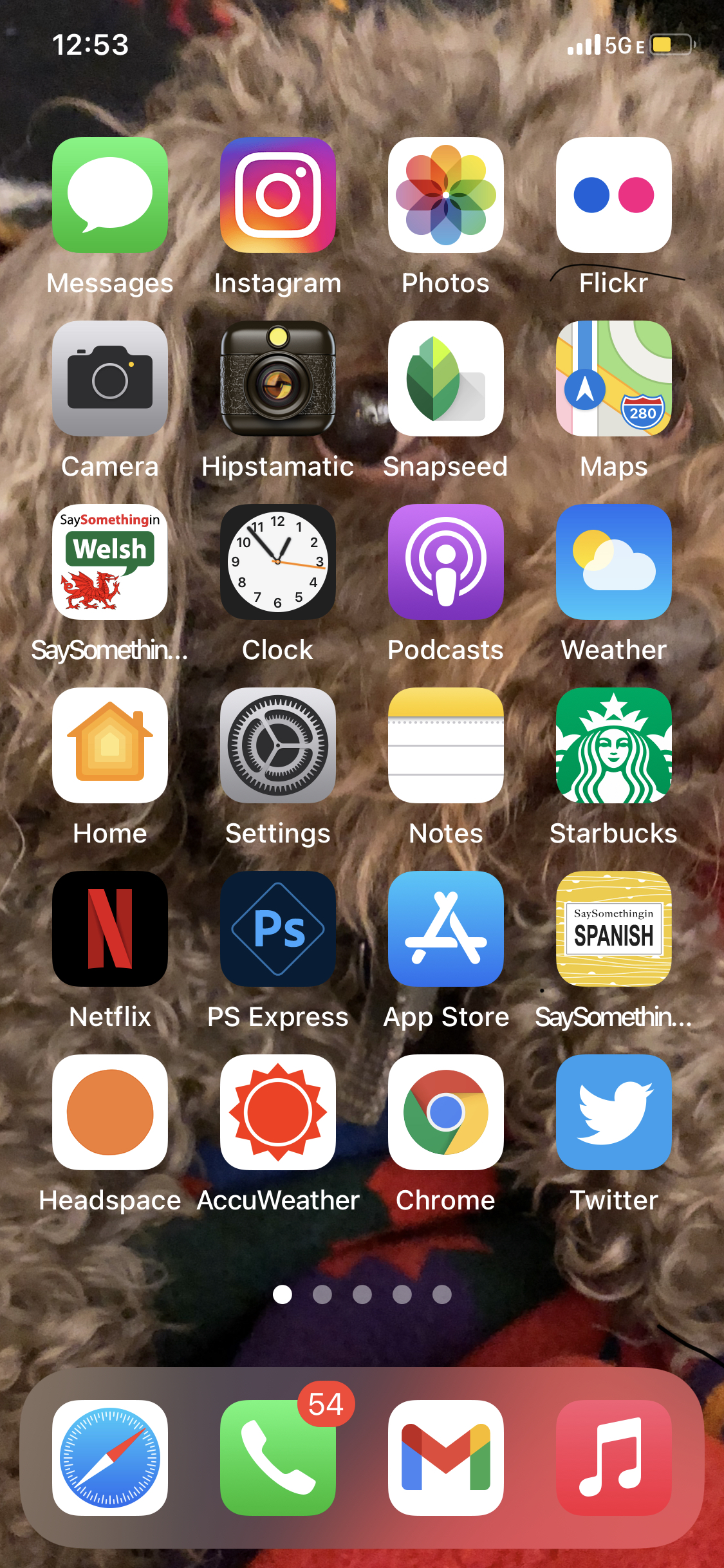Screenshot of a smartphone home screen displaying an array of apps organized into rows. The top row includes commonly used apps such as Messaging, Instagram Photos, and Flickr. The second row showcases photography-related apps like Camera, Hipstamatic (which has an icon resembling a camera), Snapseed, and Maps. Following this, the next row consists of Say Something, possibly a language learning app, Welsh (likely another translation app), Clock, Podcasts, Weather, Home, and Settings. Continuing downwards, there are apps like Notes, Starbucks, Netflix, and PS Express (identity unclear). Further down, the App Store appears along with Say Something in Spanish (another possible translation app), Headspace for meditation, AccuWeather, Chrome for browsing, and Twitter. At the bottom of the home screen, within the dock, there are four essential apps: Compass, Telephone, Gmail (Google Mail), and Music. The background image is indistinct but seems to feature a dog with lush fur.